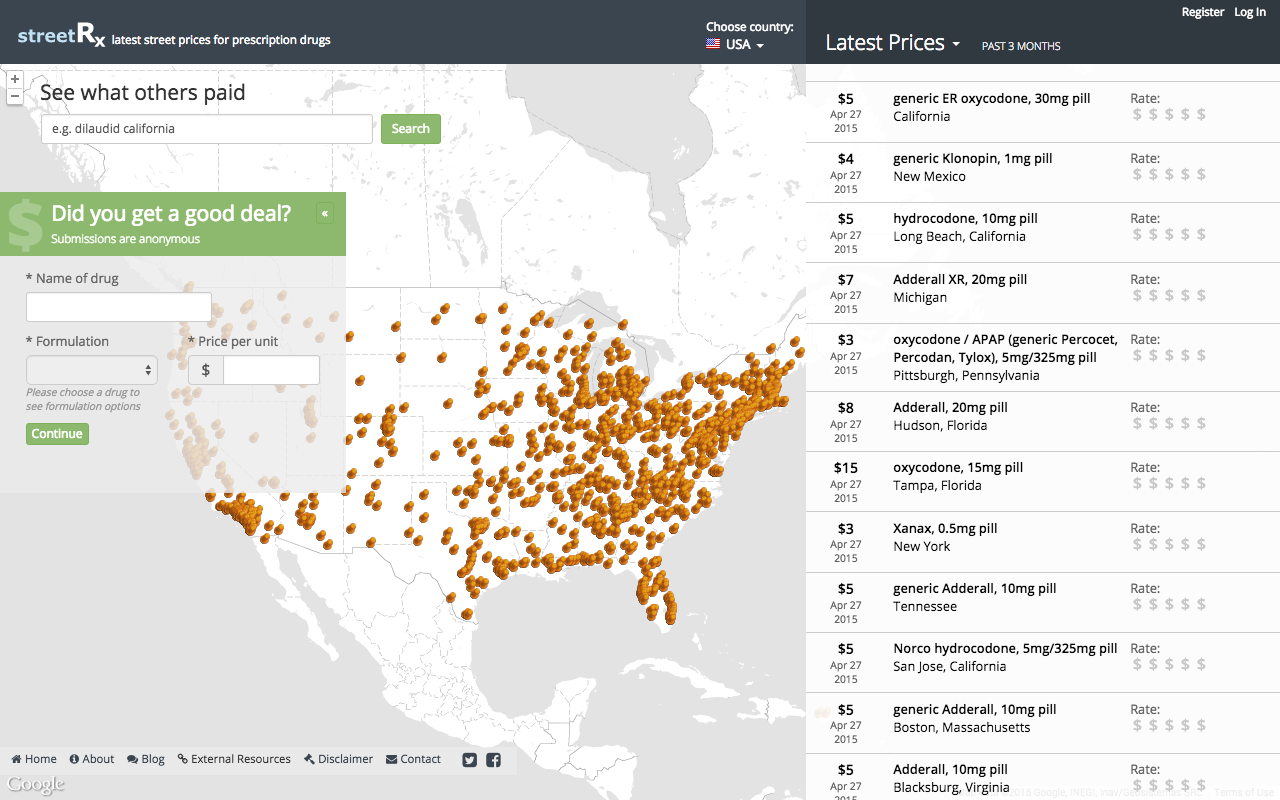This screenshot is from a website or software interface dedicated to tracking street prices of prescription drugs. At the top, there's a dark blue-gray navigation bar. From left to right, it contains the title "StreetRx: Latest Street Prices for Prescription Drugs," followed by options to "Choose Country" (with the USA preselected), view "Latest Prices" for the "Past 3 Months," and options to "Register" or "Log In."

Below the navigation bar, on the left half of the screen, there's an outline map of the United States studded with numerous orange and red dots, accompanied by the text "See What Others Paid." A search bar is present with a placeholder text, "e.g., Dilaudid, California," and a green search button. 

Beneath the map is another green button labeled "Did You Get a Good Deal? Submissions are anonymous," encouraging users to share their purchase information. Immediately below this is a column listing various prescription drugs, their formulations, and the price per unit. There's an invitation to continue exploring more prices.

Running down the left-hand side of the screen is a section titled "Latest Prices, Past 3 Months," listing various prices: $5, $4, $5, $7, $3, $8, $15, $3, $5, $5, $5, $5. Adjacent to these prices is a list of medications that includes Oxycodone, Klonopin, Hydrocodone, Adderall, and Xanax.

At the bottom of the price list, there's a rating system using $1 to $5 signs, presumably allowing users to rate the price deals they've encountered.